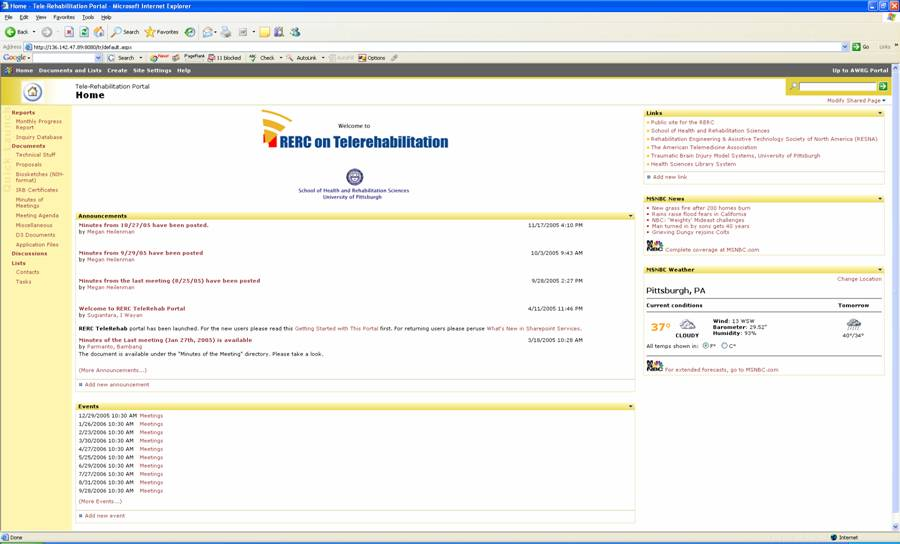The image is a screenshot of a website's homepage. At the top of the page, a banner prominently displays the text "Welcome to RERC on Tele-Rehabilitation." Directly below the banner, there's a small logo followed by some text which is illegible. On the left side of the page, a yellow navigation bar is present, featuring links in red text labeled as "export documents" and other options, though the font is too small to decipher clearly.

On the right side of the webpage, there is a vertical panel dedicated to various link sections. Among these, there is one for MNBC News and another for MNBC Weather. Below these sections, the location is identified as Pittsburgh, Pennsylvania, with current weather conditions stated as 37 degrees, suggesting a chilly atmosphere.

At the center of the page, there are more announcements displayed in red text, accompanied by four clickable links for further information. Beneath these announcements, a list of upcoming events is provided, each linked for users to click on and explore further.